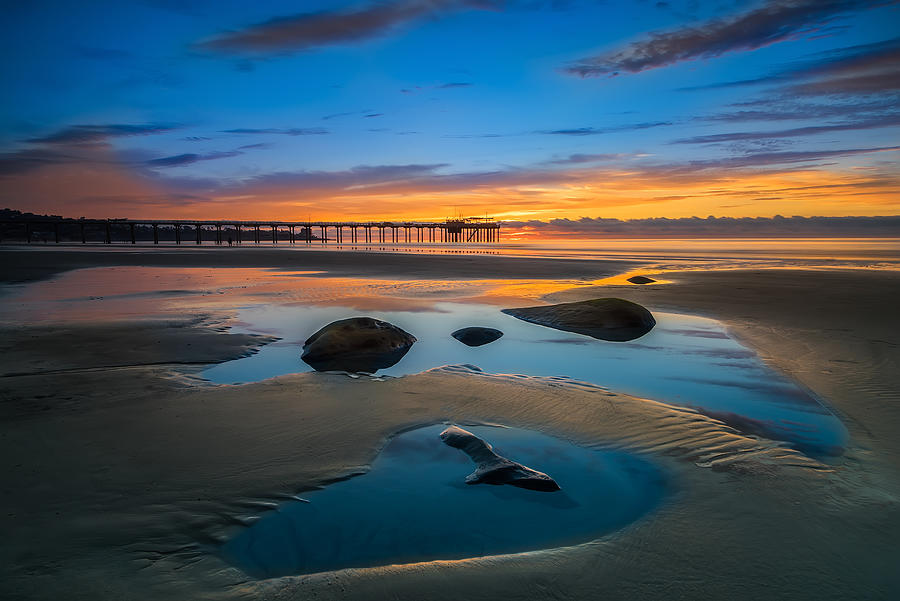The image captures a serene seaside scene at sunset, dominated by a magnificent orange and blue sky. The sun is either rising or setting, casting a golden hue over the expansive horizon, marked by a cluster of gray clouds. The foreground features a sandy shore with small pools of water left behind by the receding waves, creating a reflective surface. A wooden pier supported by stilts stretches out into the ocean, extending about halfway across the photograph, blending into the horizon. The camera's low angle accentuates the textures in the sand and the calmness of the water, adding to the tranquil ambiance of the coastal landscape.